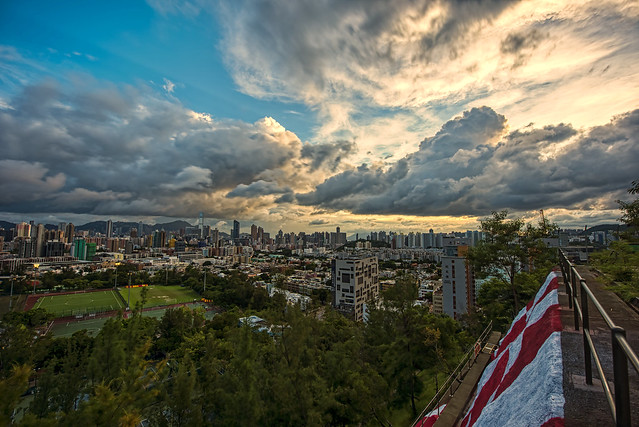A panoramic painting captures a vibrant park nestled within a bustling cityscape. In the bottom left corner, two soccer pitches surrounded by a red track are enveloped by lush green fields and dense trees. To the right of the painting, a walkway with a metal guardrail lines the edge of a significant drop, providing a safe vantage point. Below the path, a red and white banner or flag hangs at an angle, partially obscured. The cityscape in the background transitions from smaller buildings near the park to towering skyscrapers further in the distance. The sky dominates the top half of the painting with ominous grey and dark grey clouds, tinged with some blue, hinting at the sun rising or setting behind them. Far off in the distance, mountains rise to meet the sky, completing the serene yet urban landscape.